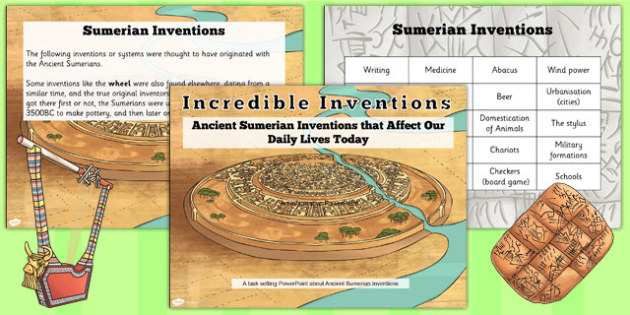The image is an artistic illustration, resembling a history book page, highlighting influential ancient Sumerian inventions. Central to the image is the caption "Incredible Inventions," followed by the phrase "ancient Sumerian inventions that will affect our daily lives today." Surrounding this central text are three sections. The left section is titled "Sumerian Inventions," listing various innovations attributed to the Sumerians, such as writing, medicine, the abacus, wind power, beer, urbanization, the stylus, domestication of animals, chariots, military formations, checkers, and schools. This section also includes a depiction of a harp adorned with a gold bull's head. The right section mirrors the left but with a different visual style, featuring a tablet with inscriptions. Details in these sections mention iconic inventions like the wheel and hint at the Sumerians' contributions to pottery-making around 3500 BC. The central image depicts a circular device, likely an ancient wheel, symbolizing the far-reaching impact of Sumerian ingenuity.